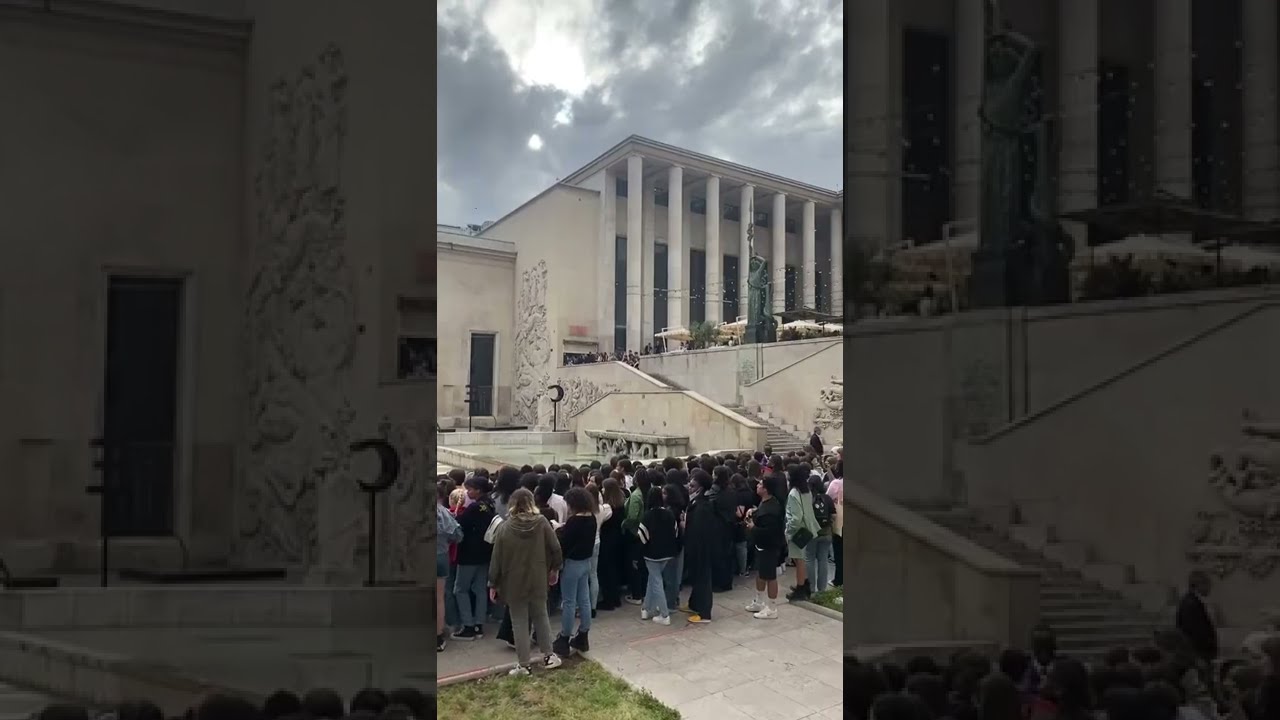The image features a detailed view of a large white building with a slightly dilapidated appearance, characterized by multiple tall cylindrical columns extending from its facade. This vertically shot cell phone image captures the main scene in the center, flanked by zoomed-in and faded sections on both the left and right sides of the frame, providing a focused close-up on the architectural details.

At the center of the building's facade, there's a roof supported by these prominent white columns. An intricately carved design is visible on the left side of the building, adjacent to a brown closed door. In front of the building, positioned from the center to the right, stands a bronze-colored statue of a woman, adding a focal point to the scene.

Below the building, a white staircase descends to a concrete sidewalk leading across the image towards the bottom right corner. Gathered in this courtyard area are approximately 50-100 people, all facing left, suggesting they are observing or participating in an event. The crowd, mostly uniform in height and mostly dressed in black shirts with blue jeans, contrasts with one individual standing on a small patch of grass in the bottom left corner, who is distinctively attired in a green suit and white shoes. Another notable figure in the bottom right of the image wears a green dress and carries a black purse.

This comprehensive caption harmonizes repeated elements from multiple descriptions, providing a vivid and detailed portrayal of the scene.